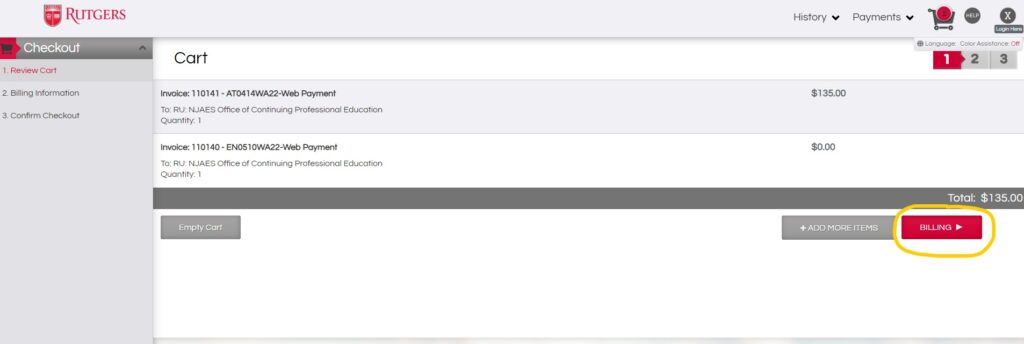A screenshot of an online checkout process is displayed from a Rutgers-themed website, indicated by a shield icon and the word "Rutgers" located in the top left corner. The process is broken down into three steps: "1. Review Cart," "2. Billing Information," and "3. Confirm Checkout." The "Review Cart" step is highlighted in red, indicating that the user is currently on this screen. 

In the cart, there are two items listed under "Office of Continuing Professional Education," both with a quantity of 1. The first item is priced at $135, while the second one is free of charge at $0. 

At the top of the screen, there are icons for exiting out, seeking help, and viewing the cart. Additionally, there are pull-down menus for viewing payment options and history. Another icon allows the user to change the language of the page.

The page shows a total amount of $135 due. Users have the option to click a button to add more items or to proceed by clicking the red button to go to the billing information screen. Notably, this red billing button is circled in yellow, indicating where to click next to continue with the checkout process.